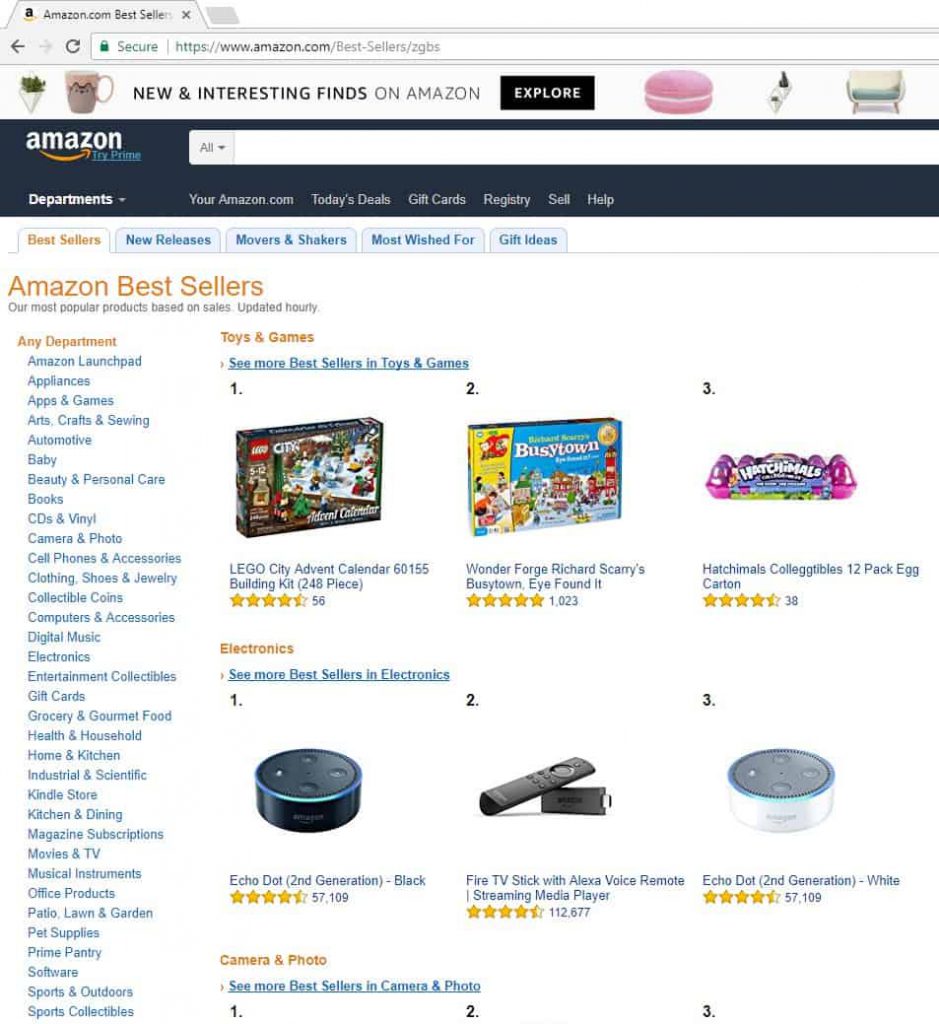**Detailed Description of the Amazon Page Screenshot**

The image is a rectangular, portrait-oriented screenshot taken from an Amazon webpage being viewed on a tablet. It lacks an outer border and is slightly taller than it is wide. The screenshot is divided into several distinct sections.

**Top Section: Tablet Browser Interface**
The uppermost part of the screenshot displays the tablet's browser interface. At the very top, there is a search bar for Amazon, distinguished by a light grey tab protruding from the left, which likely indicates it's a tablet interface. The tab features the Amazon logo, followed by the text "amazon.com: bestsellers", and an 'X' icon for closing the tab.

Below the tab, there is a standard browser header. Starting from the far left, the header includes a leftward-facing arrow that is darkened, indicating it's active, and a rightward-facing arrow that appears faded, suggesting it's inactive. Following this, there is a circular arrow icon for refreshing the page. Next to it is a long white search bar displaying a green "lock" icon, ensuring the connection is secure, followed by the URL "https://www.amazon.com."

**Main Page: Featured Items and Navigation Bar**
The main content of the Amazon page starts below the browser header. This section features a white background with five small images of items, each representing Amazon's "New & Interesting Finds" section. From left to right, the items include:
1. What appears to be a white cup with flowers and leaves inside.
2. A coffee mug.
3. An icon displaying the text "NEW & INTERESTING FINDS ON AMAZON" with "on Amazon" in lighter grey.
4. A black rectangular button labeled "EXPLORE" in white, all caps.
5. A pink object that resembles either a pillow, a cookie (macaroon), or a smart speaker button.
6. An image of an unrecognizable small object.
7. A two-seat loveseat.

Beneath this featured section, there is a navigation bar with a black background, showing the Amazon logo in the top left corner accompanied by a white search bar on its right. The search bar on this navigation panel is empty.

**Navigation Links and Category Tabs**
Next, the screenshot shows a series of navigation links on the left side in bold white font under the label "Departments." The links include:
- YourAmazon.com
- Today's Deals
- Gift Cards
- Registry
- Sell
- Help

To the right of these links, there is an empty area. Further below, the page has five tabs, with the leftmost tab labeled "Best Sellers" in orange, indicating it is selected. The other tabs are:
- New Releases
- Movers & Shakers (with an ampersand)
- Most Wished For
- Gift Ideas

**Main Content: Amazon Best Sellers**
The main content area prominently displays "Amazon Best Sellers" in large orange font, followed by a description in smaller font stating, "Our most popular products based on sales, updated hourly."

This section is split into two main columns:
- The left column (about 25% of the width) lists various departments in blue text, categorized under "Any Department." The departments include Amazon Launchpad, Appliances, Electronics, Digital Music, Sports Collectibles, and others.

- The right column showcases the best-selling products, divided into two rows of three products each. 

**Top Row: Toys and Games**
1. **LEGO City Advent Calendar:** Image of the box, 4.5 stars rating, 56 reviews.
2. **Wonder Forge Richard Scarry's Busy Town, Eye Found It:** Game box image, 5 stars rating, 1023 reviews.
3. **Hatchimals CollEGGtibles 12-Pack Egg Carton:** Egg carton image, 4.5 stars rating, without specific review count visible.

**Bottom Row: Electronics**
1. **Echo Dot (Black):** Image of the black Echo Dot, 4.5 stars rating.
2. **Fire TV Stick with Alexa Voice Remote:** Image of the Fire TV Stick, 4.5 stars rating, 112,677 reviews.
3. **Echo Dot (White):** Image of the white Echo Dot, 4.5 stars rating.

The very bottom of the image slightly cuts off the third section labeled "Camera & Photo," showing partial numbers "1, 2, and 3" but no product images.